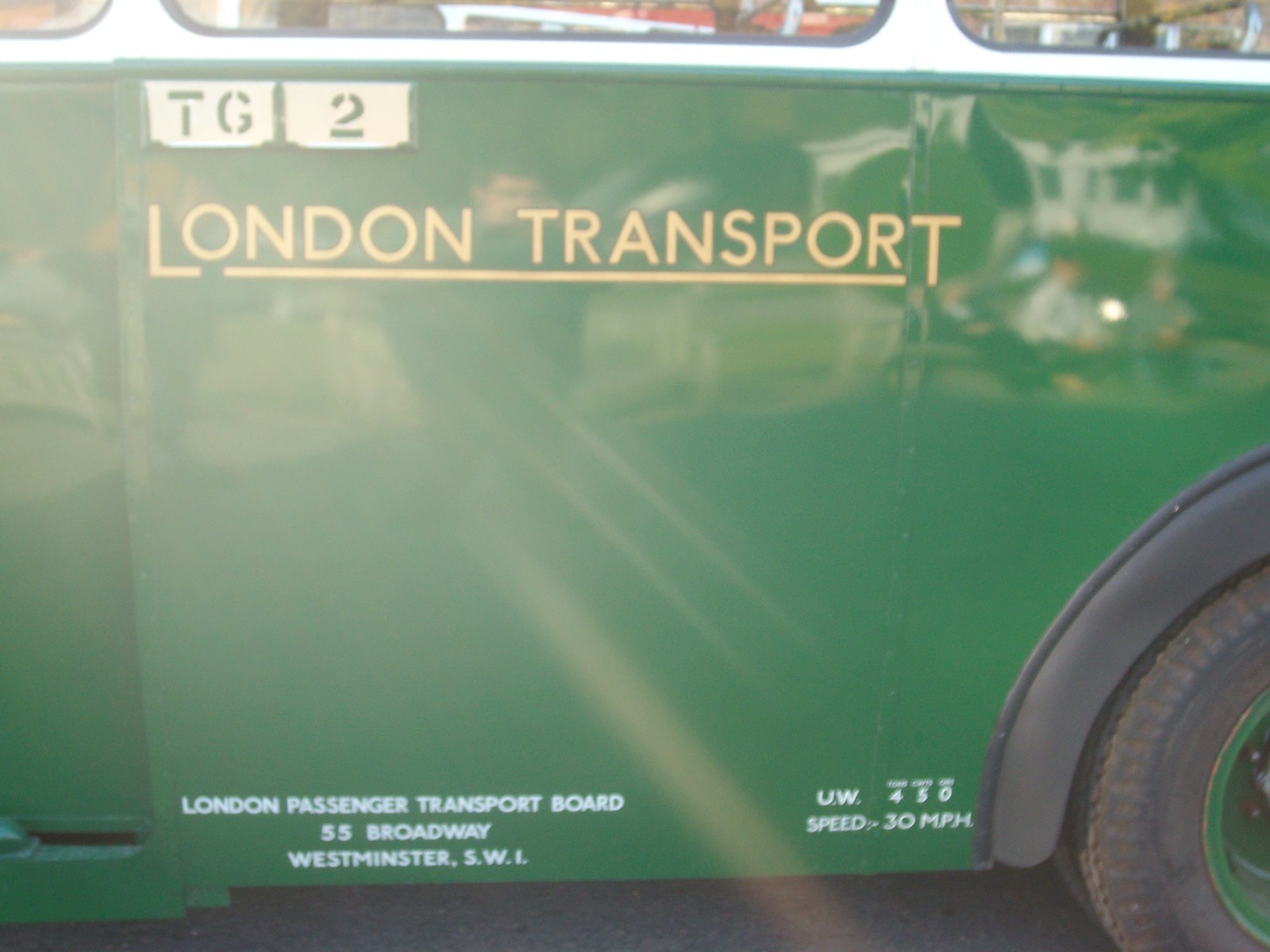Close-up view of the side of a green public transport vehicle, possibly a bus or truck. The side paneling prominently displays the ID number "TG2" at the top left. Below this, in yellow lettering, the text reads "London Transport" with an underline beneath the words. At the bottom of the panel, near the baseboard, small white text details "London Passenger Transport Board, 55 Broadway, Westminster, SW1." Additionally, in smaller text on the right side, it reads "UW450, Speed 30mph." The top of the vehicle shows part of a window with a white frame, and visible at the bottom right corner is a tire with a green hubcap and black rubber forming a half-moon shape above it.